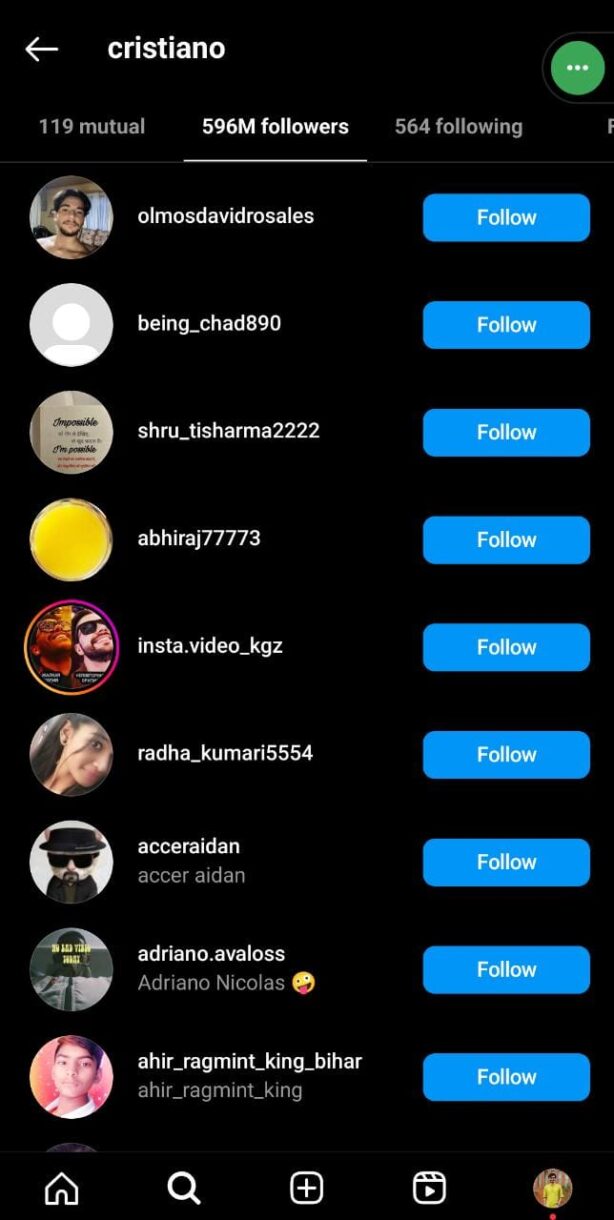This is a detailed caption describing a screenshot of an Instagram app interface. 

The screenshot showcases various statistics related to an individual's profile. Highlighted against a black background, the text appears in white font for clear visibility. On the left side of the screen, there are small circular profile images, each paired with corresponding text. 

The interface lists the total number of followers the person has, the mutual followers shared between the user and these profiles, and the number of people the user is following who also have Instagram accounts. A small circular profile picture representing the person's social media identity is prominently displayed. 

To the far right of each profile entry, a blue "Follow" button indicates potential followers that the user can choose to follow. In this particular screenshot, there are nine such profiles presented. 

At the bottom of the screen, navigation icons are neatly aligned and centered, providing quick access to various Instagram functions such as the home page, search, post creation, and Instagram Reels. The entire layout is clean and focused, with no additional subtle details beyond those described.